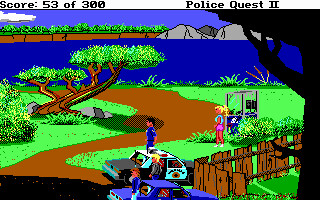Screenshot from a classic vintage-style game, resembling old-school arcade visuals. The image is characterized by its 2D pixelated and fuzzy graphics, typical of retro games, and is notably smaller compared to modern screenshots or photos.

A white banner at the top displays game information: on the left, "Score: 53 of 300" is written in black, and on the right, the title "Police Quest II" appears. Below this banner, the game scene unfolds.

In the game, a police car is parked to the left, with a purple-blue car to its right. Outside the cars, a policeman stands on a pixelated patch of grass next to a brown paved walkway. He is accompanied by another figure standing behind him near a payphone area, which is surrounded by bushes.

In the background, a serene lake lies with poorly drawn, pixelated mountains to the right, under a blue sky with a single cloud in the top left corner. To the left of the policeman, a curved tree grows diagonally to the right with branches that sprout vibrant green leaves, positioned on a patch of grass adjacent to the walkway.